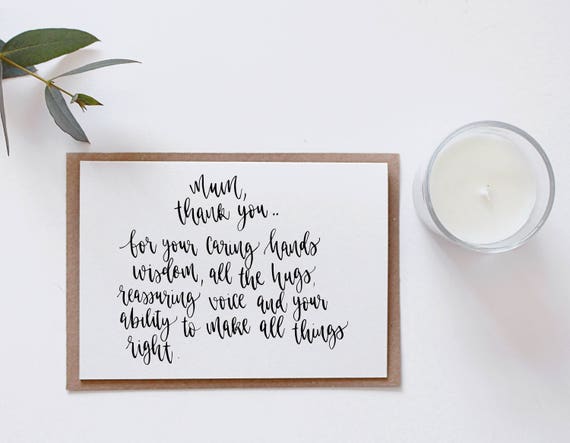The image depicts a peaceful and serene tribute to motherhood, captured from a top-down perspective. At the center lies a rectangular white plaque bordered by light brown, adorned with elegant black cursive text that reads, "Mom, thank you for your caring hands, wisdom, all the hugs, reassuring voice, and your ability to make all things right." To the right of the plaque is an unlit white candle sheltered in a clear glass holder, adding to the tranquil atmosphere. In the upper left corner, a green leaf peeks into the frame, hinting at the presence of a plant just outside the shot. The setup rests on a white surface that enhances the purity and simplicity of the scene.